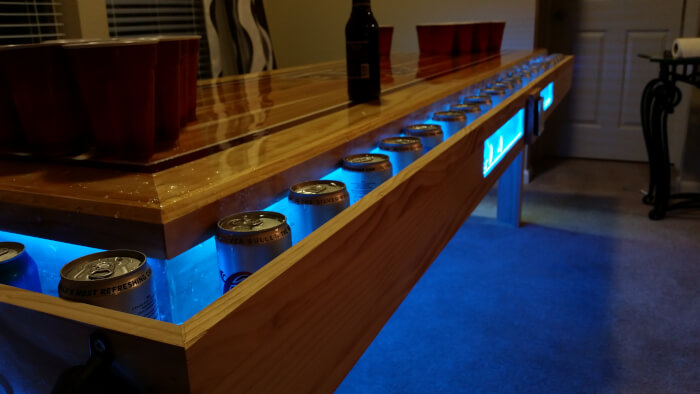This indoor photograph showcases a custom-made wooden bar table emanating a striking DIY aesthetic. The rectangular wooden bar, finished with a natural varnish, spans the bottom left to the top of the image. Across its surface, there are red Solo cups and a central dark brown beer bottle. The table features a unique drop-down pocket running its perimeter. Inside this pocket, illuminated by a blue light, numerous beer cans with gold tops and white sides (likely Coors) are neatly arranged, suggesting a built-in chiller function. The floor beneath the table may appear bluish from the light reflection or feature a blue rug. To the far right, a white household door and a small dark brown table with paper towels enhance the impression of a cozy home bar setup. The overall color palette predominantly features natural browns and blues, complemented by touches of red, white, and gray, with no visible text in the image.